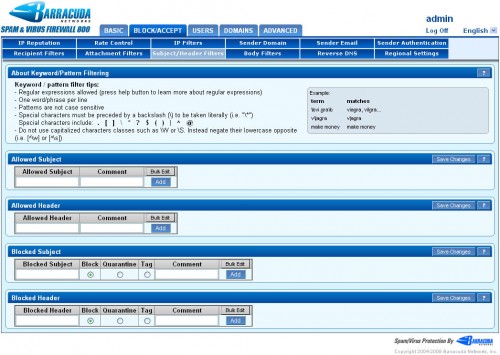A webpage filled with numerous blue brackets catches the eye. The prominent text on the page reads, "Barb Borrowed." Given the design elements and terminology, it appears to be a scuba diving-related website. The usage of brackets might indicate a coding interface, possibly intended for booking or scheduling scuba diving sessions, or a decorative element typical of a tech-savvy design.